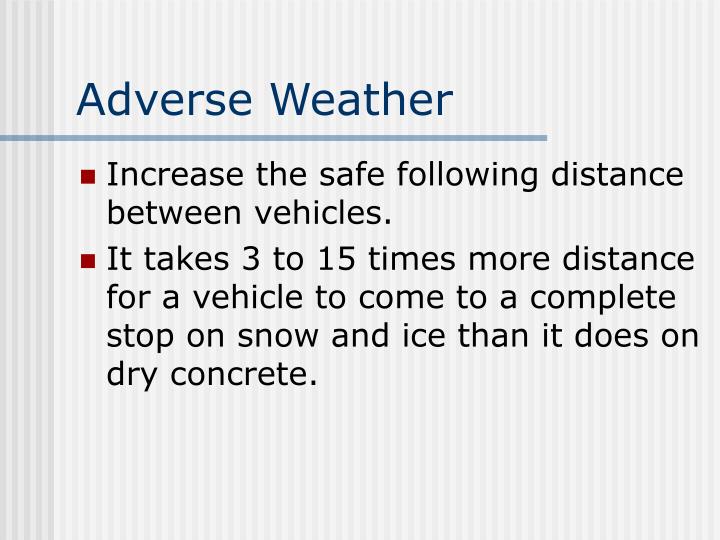The image is a graphic resembling a PowerPoint slide or informational display with a white background featuring thin gray stripes. The title at the top reads "Adverse Weather" in blue letters, underlined by a dark gray line. Below the title, the content is organized with two red square bullet points. The first point advises to "increase the safe following distance between vehicles." The second point states that "it takes 3 to 15 times more distance for a vehicle to come to a complete stop on snow and ice than it does on dry concrete." The text is in black, and additional darker gray lines are present on the left side of the image.